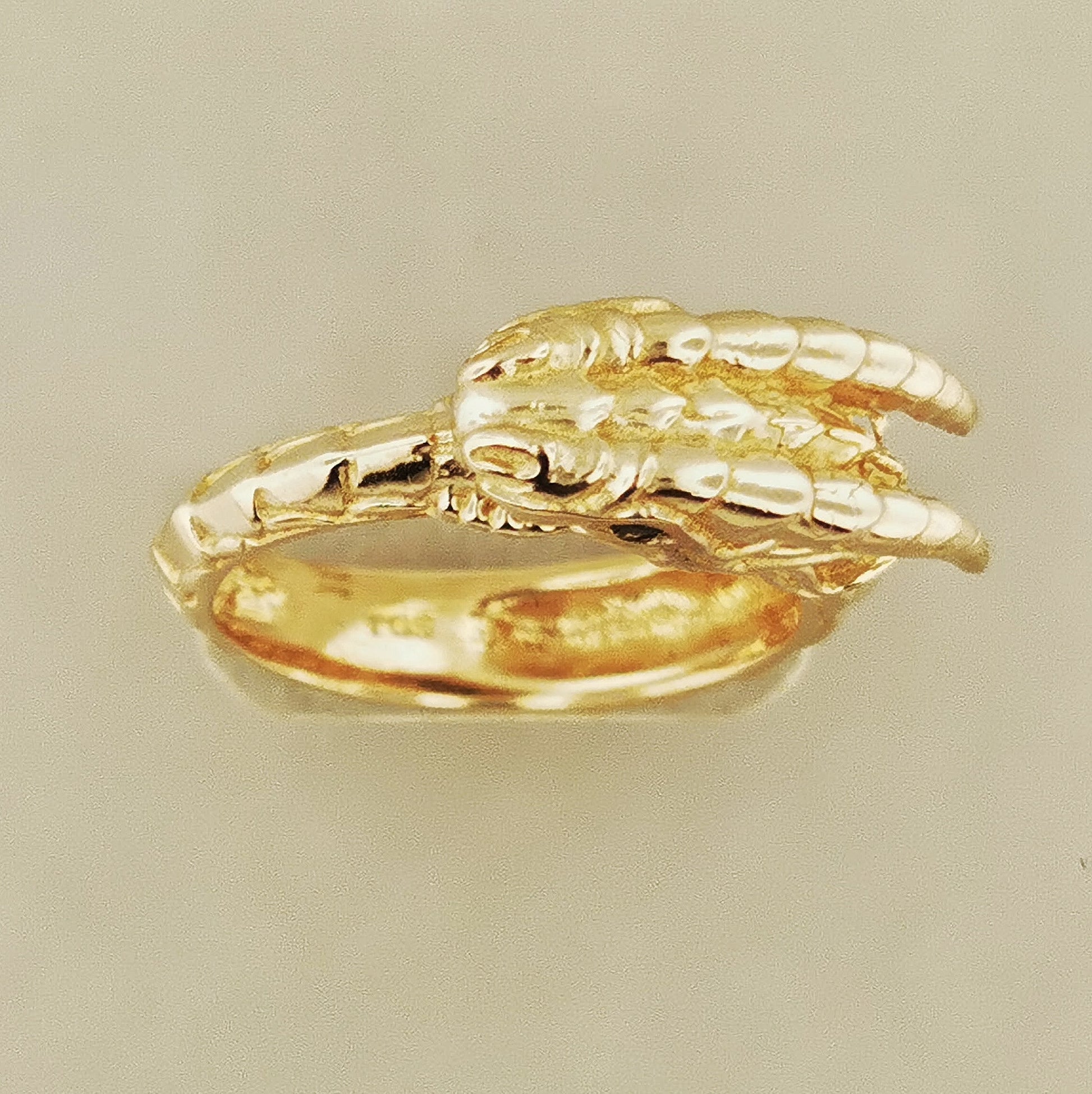This is a close-up photograph of an exquisite piece of jewelry known as the Eternal Dragon Ring. Crafted from 24-karat gold, this thick, circular ring is intricately designed to resemble a dragon with remarkable detail. The dragon motif features detailed scales and pronounced double-angled horns, which are mirrored on either side of the piece. The top of the ring displays exquisite indentations, enhancing its ornate appearance.

This captivating ring portrays a dragon that appears to be swallowing its own tail, thus forming a continuous, golden loop. The head of the dragon, crafted with delicate precision, includes two nostrils that flawlessly transition into the double horns. A keen eye can notice a single, exquisite cubic zirconia (CZ) eye partway down on the left side of the band, adding a touch of brilliance to the design. Positioned against a beige background, the intricate details of this ring, from its scales to its horns and eyes, are brought to life, showcasing why it has earned the moniker the "Eternal Dragon Ring."